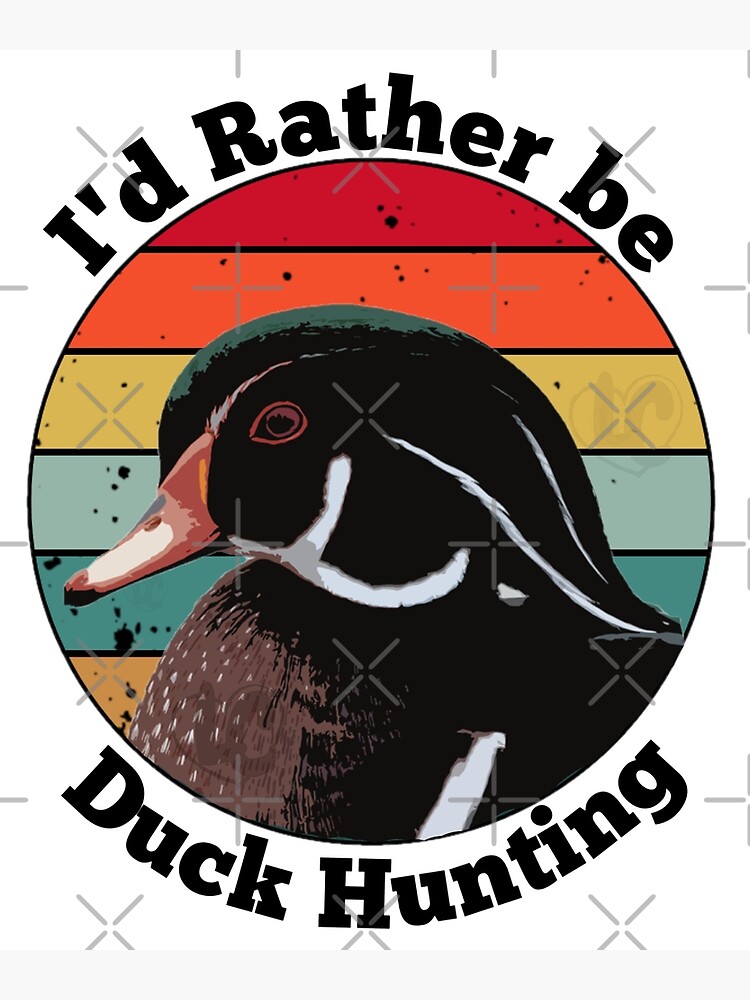This is a detailed drawing designed for potential T-shirt printing, featuring a central depiction of a duck within a circular frame. The circle is outlined in black and adorned with the text "I'd rather be duck hunting." The phrase is arched, with "I'd rather be" positioned at the top and "duck hunting" at the bottom. Inside the circle, the background comprises horizontal slats resembling wood in vibrant hues of red, orange, yellow, light blue, teal, and darker orange. The duck, situated in front of this multicolored backdrop, is intricately rendered with a green head, white stripes extending from the back of its head, and a brown and white beak. Its chest features white spots on a brown body, with additional white feathers extending from its belly towards the center. The overall composition includes watermarks and measuring lines, giving it a preparatory look for apparel design. The duck's head, characterized by its round shape, faces towards the left, completing the detailed and colorful presentation.